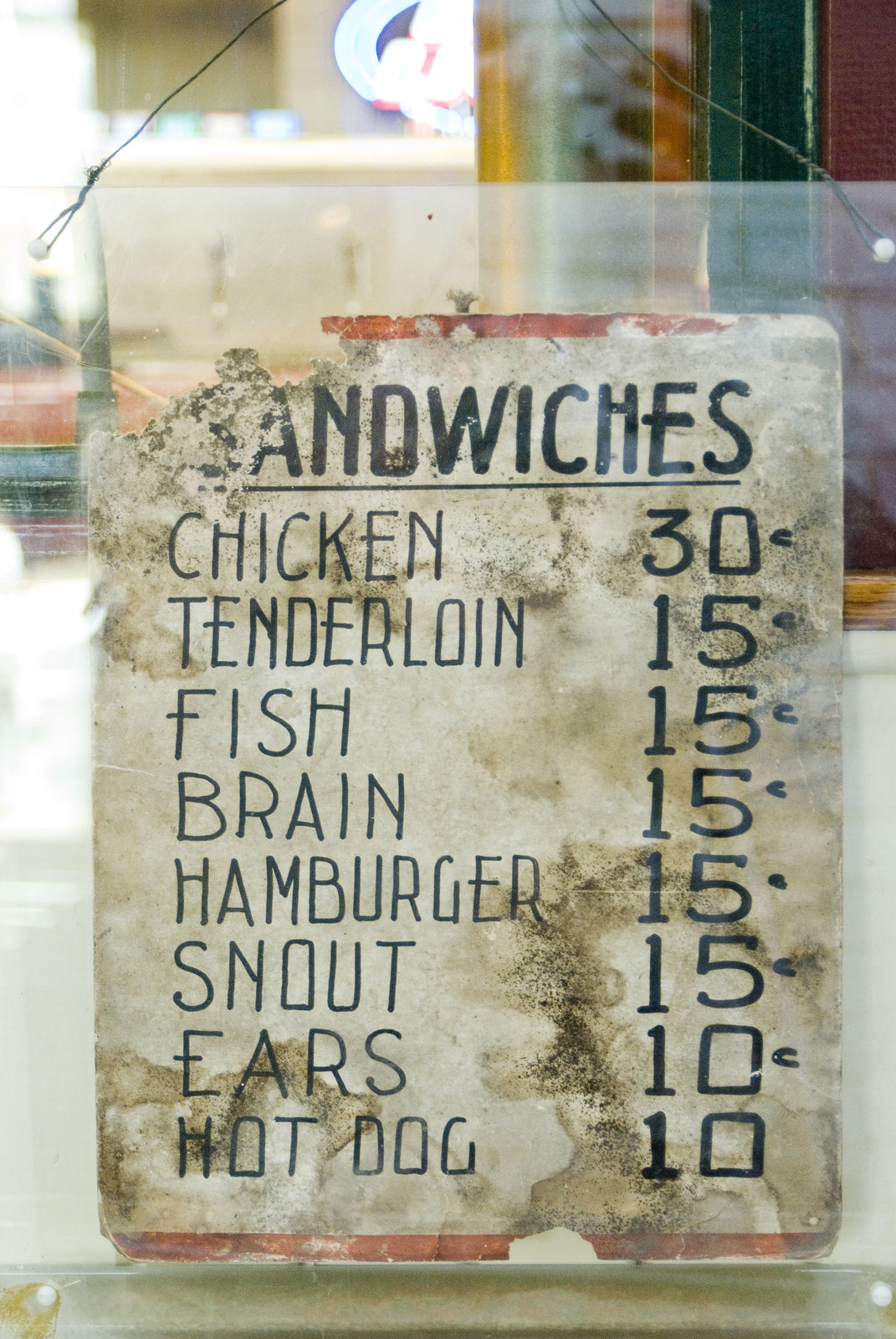A weathered and dirty white sign, emblazoned with the word "andwiches" (missing an 'S' due to wear), serves as the menu for a modest eatery. Written in black text are various food items and their prices, likely in cents, although the currency is uncertain. The menu lists:

- Chicken: 30¢
- Tenderloin: 15¢
- Fish: 15¢
- Brain: 15¢
- Hamburger: 15¢
- Snout: 15¢
- Ears: 10¢
- Hot Dog: 10¢

A prominent red line borders the top and bottom of the menu, which is affixed to a piece of clear plexiglass suspended by wires. The sign has visible water and dirt stains, indicating exposure to the elements or prolonged use. Beneath the word "andwiches," a long black line underscores the deteriorated text, hinting at the establishment's focus on sandwiches despite the condition of the signage.